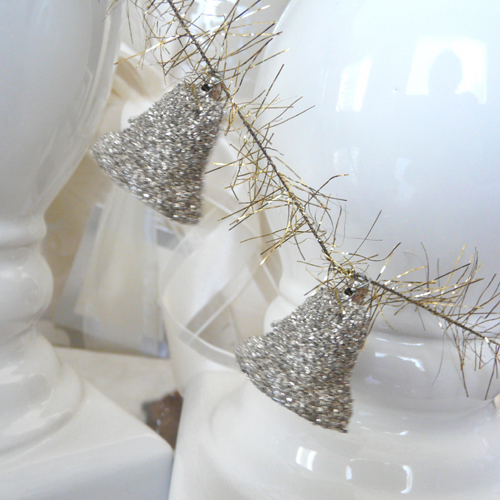This is a close-up, color photograph showcasing a festive decoration. The primary focus is on a taut string resembling tinsel, adorned with thin, stringy gold leaf ribbons. Hanging from this string are two small, ornate bells that appear to be covered in a highly reflective material, similar to tinsel or sequins, adding a shimmering effect to the scene. The first bell hangs slightly higher than the second, both connected along the string that stretches diagonally from the upper left to the bottom right of the image. The background is blurred but reveals white porcelain objects, possibly vases, with ridge details, and a hint of lace-like material draped behind the bells, enhancing the overall decorative aesthetic.